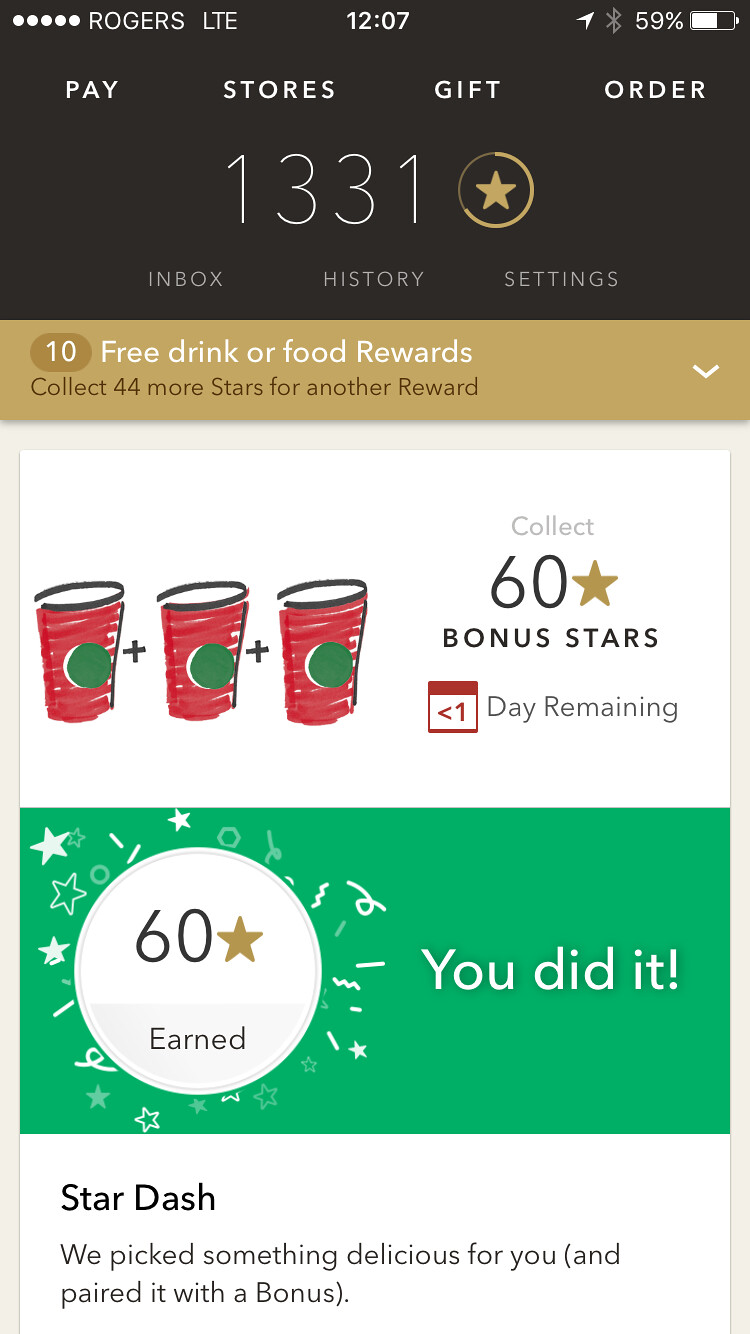This screenshot from a phone displays a coffee rewards program app, under the Rogers LTE network, taken at 12:07 with 59% battery life remaining. The app interface is organized into four sections. At the top, a black box containing tabs labeled "Pay," "Store," "Gift," and "Order" is visible. Below this, the user’s current point total is prominently displayed in black text as "13.31 points," along with "10 free drink or food rewards" and a prompt to "collect 44 stars for another reward." The second section features an image of three red coffee cups with the note that "3 coffee mugs equal 60 stars," and highlights a remaining one-day opportunity to collect 60 bonus points. The third section is green, celebrating the earned "60 stars" with the words "You did it" inside a circle adorned with stars and squiggly lines. The final section, labeled "Star Dash" in white text, proclaims, "We picked something delicious for you and paired it with a bonus." At the bottom of the screen is a mention of a website link: "www.microsoft.com."